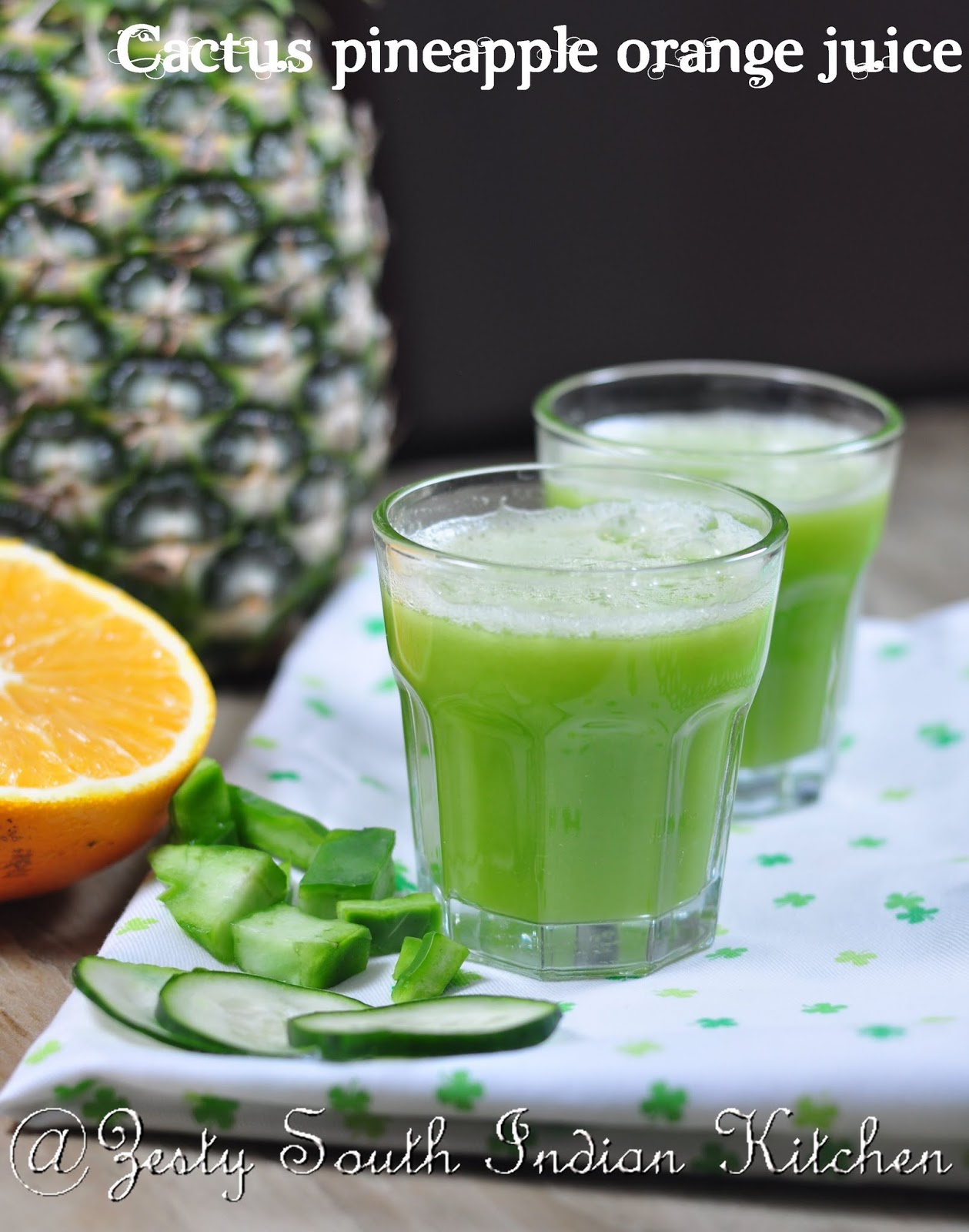The image is a color photograph in portrait orientation featuring an advertisement for a company. The subject of the photograph prominently displays two lowball whiskey glasses filled with a frothy green juice, presumably flavored with cactus, pineapple, and orange. These glasses are positioned on a white tablecloth adorned with green clover leaf designs, hinting at a festive theme, possibly St. Patrick's Day. Surrounding the glasses are several slices of cucumbers and pieces of chopped cactus on the left, half of an orange further to the left, and a mostly visible but partially cropped green pineapple in the left background. The background at the top of the image is black, providing a stark contrast to the vivid colors of the fruits and the green juice. Across the top of the image, there is white text that reads "Cactus Pineapple Orange Juice," while the bottom features script text that says "Zesty South Indian Kitchen," likely the name of the company being advertised.